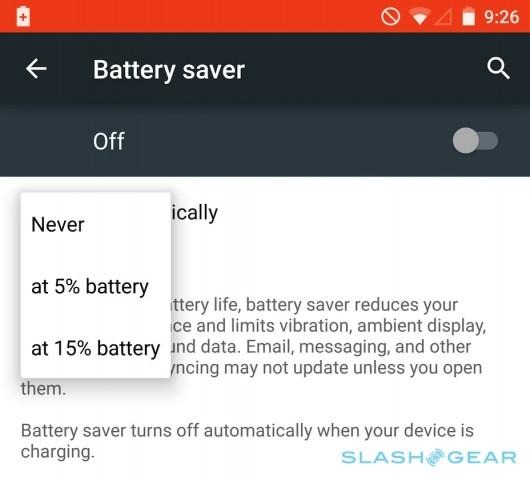In this image, there is a screenshot taken from a smartphone. In the upper left-hand corner, we see a unique battery icon with a plus sign inside it. On the upper right-hand corner, the displayed time is 9:26. Adjacent to the time is another battery icon which appears to be nearly full. The phone shows no service bars, and the Wi-Fi signal indicates two filled sections. Next to the Wi-Fi symbol, there is an icon of a circle with a line through it. 

On the left side, just below these icons, the text "Battery saver" is visible alongside a back button, symbolized by a left-pointing arrow. On the right side is a search icon. Beneath this section, the word "Off" appears with a toggle switch indicating that the battery saver is currently off.

Below this interface, there is a pop-up message on the left side. The message reads “Never” at 5%, 10%, or 15% battery, and the partial text beneath it includes a paragraph explaining the battery saver function: "Battery saver reduces your… Limits vibration, ambient display…" The text is cut off but mentions that email, messaging, and other applications may not update unless opened. Additionally, it states, "Battery saver turns off automatically when your device is charging,” though the remaining part of the paragraph is obscured.

The descriptive caption would be suitable for providing readers with a clear and highly detailed understanding of the screen's layout and the information presented.